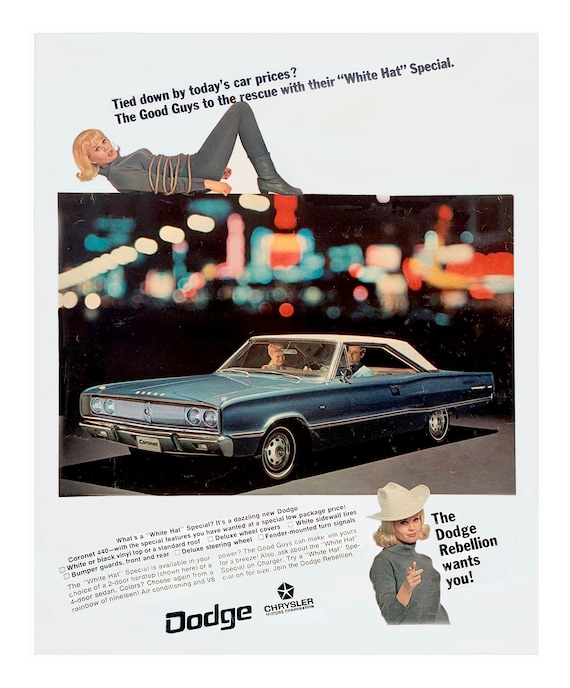This retro magazine clipping advertisement for Dodge Chrysler showcases a dazzling blue Dodge Rebellion with a distinctive white hood. Set against an off-white background, the central image features a couple in the car, parked on a paved surface with a scenic nighttime city backdrop. Above them, a blonde woman with a bob haircut, dressed in a gray turtleneck, pants, and boots, is tied up with rope and lying on her back, symbolizing being "tied down by today's car prices." The text above her reads, "Tied down by today's car prices? The good guys to the rescue with their white hat special." In the lower right corner, the same woman appears again, now untied and sporting a white cowboy hat, pointing at the viewer, accompanied by the slogan, "The Dodge Rebellion wants you." Below this, detailed text promotes the White Hat Special, highlighting the Dodge Coronet 440 and its attractive features, such as a wider black vinyl top, deluxe wheel covers, and fender-mounted turn signals. The advertisement concludes with the Dodge and Chrysler logos.